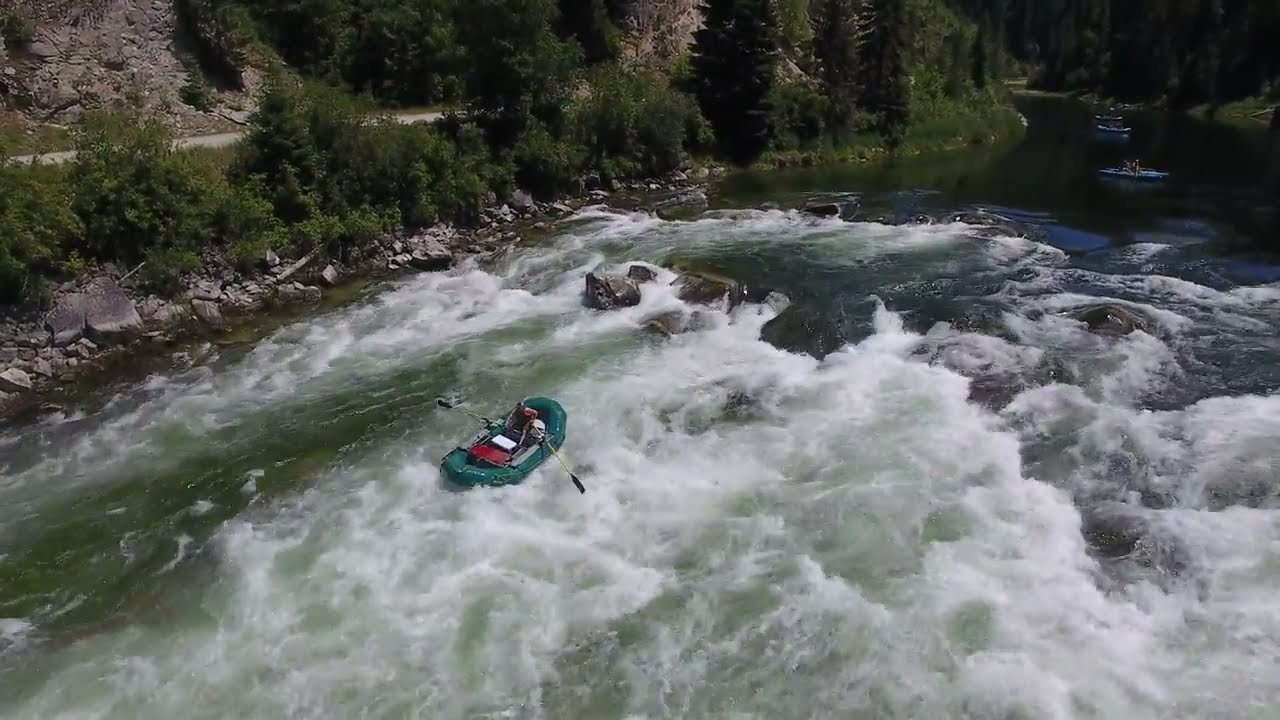The image captures a blue raft navigating through a rugged river, characterized by churning, frothy white rapids. The raft, composed of two light blue cylindrical pontoons and a main square body, carries three individuals who have their backs turned to the camera. One is distinctly dressed in a combination of yellow, red, and white. Another person is identifiable by a white coat and hat. A paddle dangles in the water while another is held aloft, indicating the effort required to steer through the turbulent flow. The river itself transitions from wild, rapid-filled waters to calmer, flat sections further downstream. Flanking the river are grayish-beige rocks interspersed with vegetation, and alongside, at a higher elevation, runs a road with a white car seen in the distance with its back door open. The landscape is encased in a canyon or valley with a rocky cliff on one side adorned with greenery, creating a vivid scene of adventure amidst natural beauty.